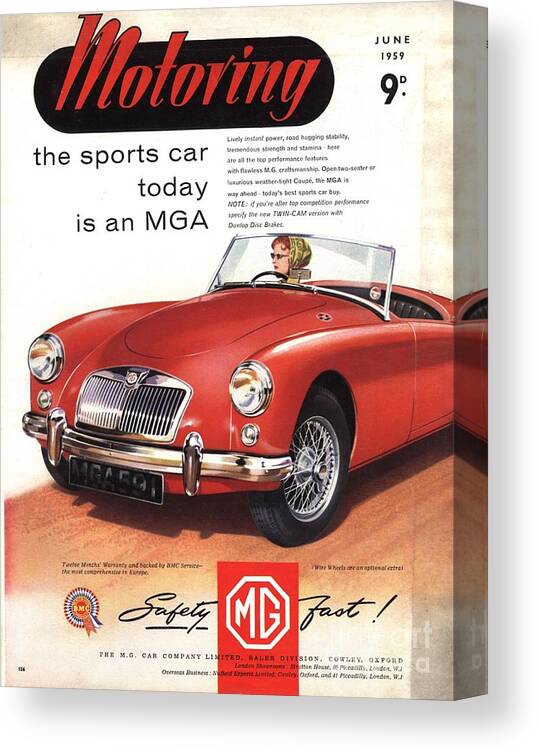This is an advertisement poster from June 1959, likely featured in an automobile magazine. At the top, a black banner hosts the red font text "MOTORING." In the upper right corner, it reads "June 1959, 9D," on the left of which is "The sports car today is an MGA" in black font, followed by a descriptive paragraph. The centerpiece is an illustrated red convertible sports car with distinctive wire wheels and chrome accents, being driven by a woman with red hair, sunglasses, and a headscarf. The steering wheel is on the right side, indicating its British origin, supported by a British-style license plate. The car faces slightly left, with the woman gazing in that direction from behind the glass windshield. The lower portion of the poster features the phrase "Safety Fast" in stylized cursive. Below this, within a red octagonal shape, the letters "MG" are prominently displayed, marking the car as part of the MG (Morris Garages) brand. The overall color palette includes black, red, off-white, light green, silver, and gray. The image beautifully captures the sleek design and allure of the MGA sports car in the late 1950s.